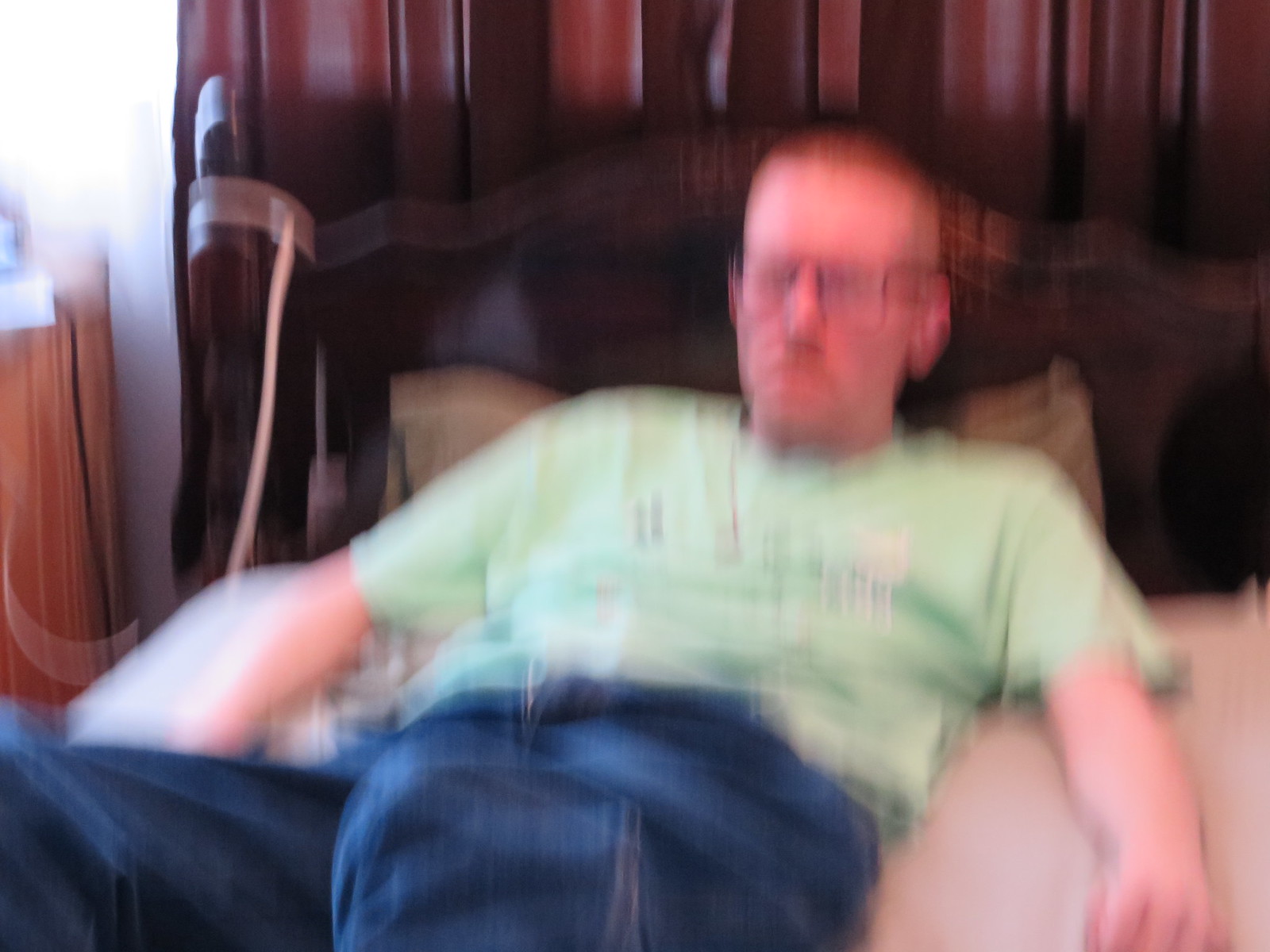This is a very blurry, out-of-focus photograph of a young white man positioned centrally and reclining on a bed. The man, who is likely asleep or resting as he reclines, has very short brown hair and is wearing dark brown-rimmed glasses. He is dressed in a light green T-shirt, possibly featuring some drawings or graphics on the front, and a pair of blue jeans with his legs extended. His left and right arms are visible, although his right hand is out of frame. He is lying on a bed with beige or tan bed covers, partially supported by a brown pillow, with a dark brown wooden headboard visible behind him. To the left of the image, there is what appears to be a cane or similar long, brown object, as well as a glimpse of a brown desk or furniture piece just out of frame.